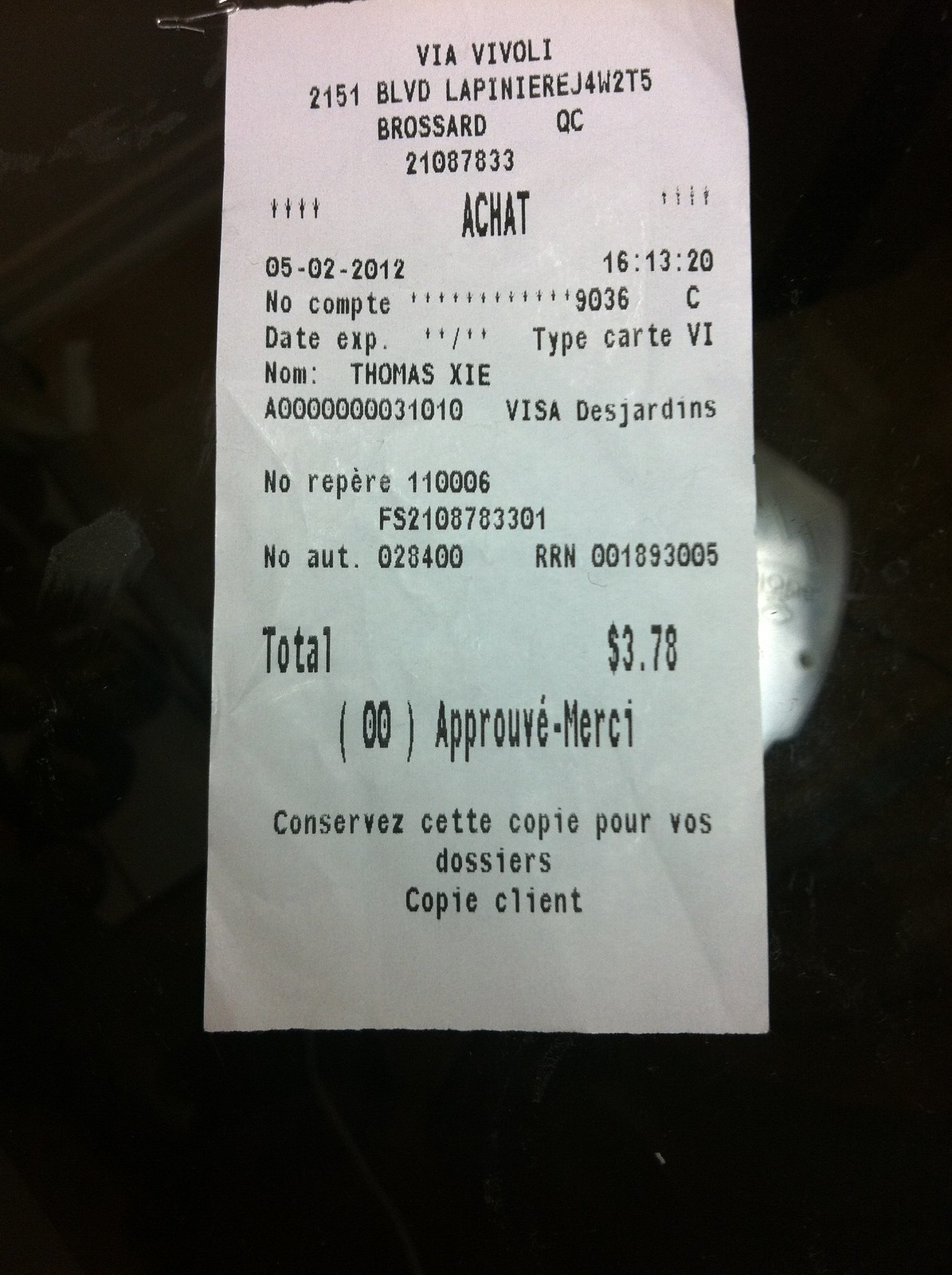This is an image of a receipt with a white background and black text. The receipt is from a business named "Via Vivoli," located at 2151 Boulevard Lapineer, J4W 2T5 in "Rosterd" QC, likely referring to Quebec City, Canada. The receipt number is 21087833. It includes the following transaction information: the purchase was made on May 2, 2012, at 4:13 PM and 20 seconds. The payment was processed using a Visa credit card with an obscured number and an expiration date mentioned but not visible in the image. The cardholder’s name is Thomas XIE. Portions of the receipt text appear to be in French.